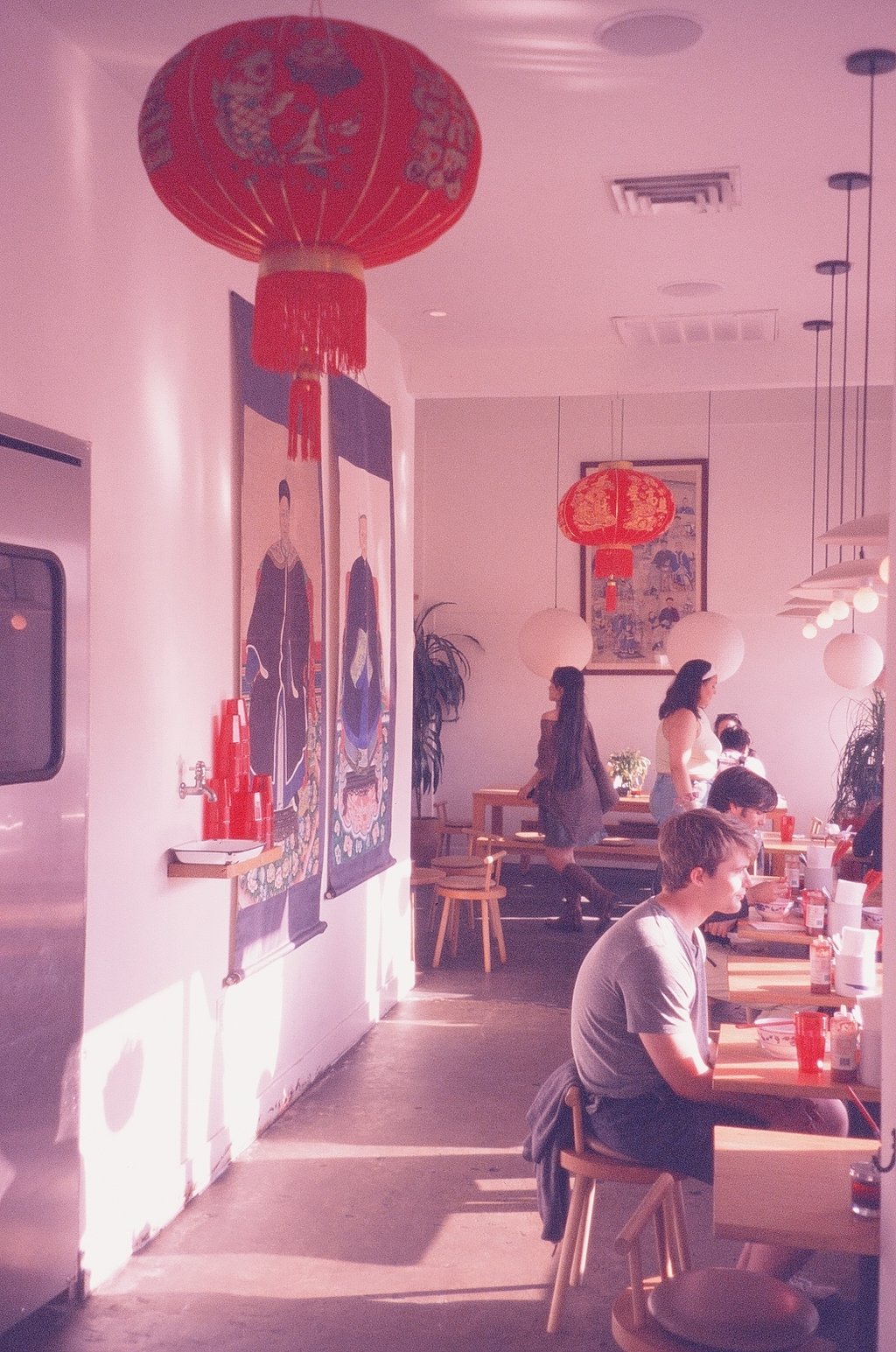This photograph depicts the interior of an Asian restaurant bathed in daylight, with sunlight streaming in and illuminating the scene. The room is adorned with traditional art on the walls and paper lanterns, both red and white, hanging from the white ceiling. The walls are also white, contributing to a bright and airy atmosphere. The dining area features light brown wooden chairs and tables arranged throughout the space. 

There are seven people visible in the scene: two men sitting at different tables enjoying their meals, two women standing – one walking towards the dining area and another across the room – and a few more people seated at a distant larger table. The patrons are using red cups and bowls, adding to the primarily red, white, and black color scheme of the restaurant. 

In the background on the left, a chrome service door with a window at the top leads to a long hallway. The scene also includes two large posters depicting regal figures adorning the walls, though their details are somewhat obscured by the angle. 

Overall, the restaurant's interior exudes a traditional and inviting ambiance, accentuated by the combination of cultural decorations, warm wooden furnishings, and the bustling activity of its patrons.